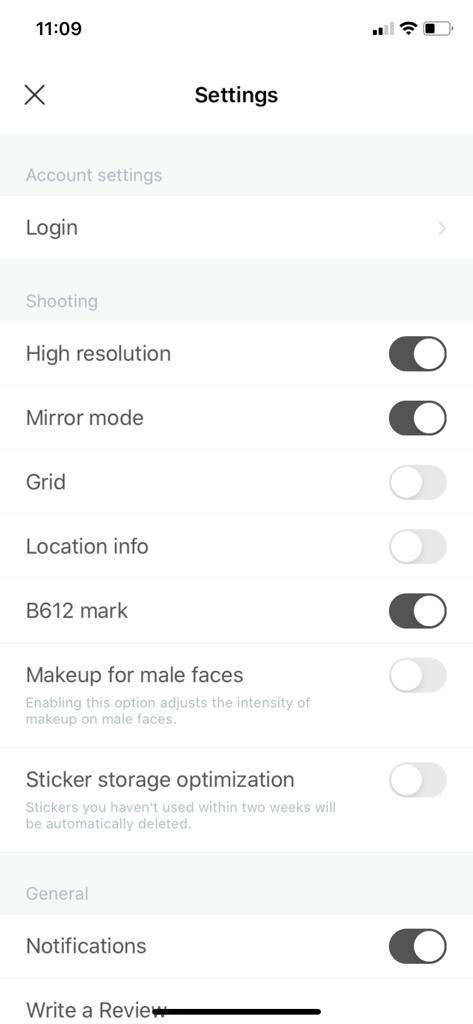Screenshot of an app's settings menu with detailed user options. 

1. **Settings Overview**:
   - Settings icon with an "X" icon next to it.
   - Several main categories, including "Account Settings," "Shooting," and "General," each highlighted with a gray rectangle.

2. **Account Settings**:
   - "Log in" option visible.

3. **Shooting Settings**:
   - "High Resolution" setting toggled ON (circle to the right and shaded).
   - "Mirror Mode" setting toggled ON (circle to the right and shaded).
   - "Grid" setting toggled OFF (circle to the left).
   - "Location Info" setting toggled OFF (circle to the left).
   - "B612 Mark" setting toggled ON (circle to the right and shaded).
   - An option to apply "Makeup for male faces," with a description: "Enabling this option adjusts the intensity of makeup on male faces."

4. **Sticker Storage Optimization**:
   - Description: "Stickers you haven't used within two weeks will be automatically deleted."

5. **General Notifications**:
   - General notification setting toggled ON (circle to the right and shaded).
   - An option to "Write a Review" available.

Some settings names and options are shaded, indicating they may be currently selected or highlighted.